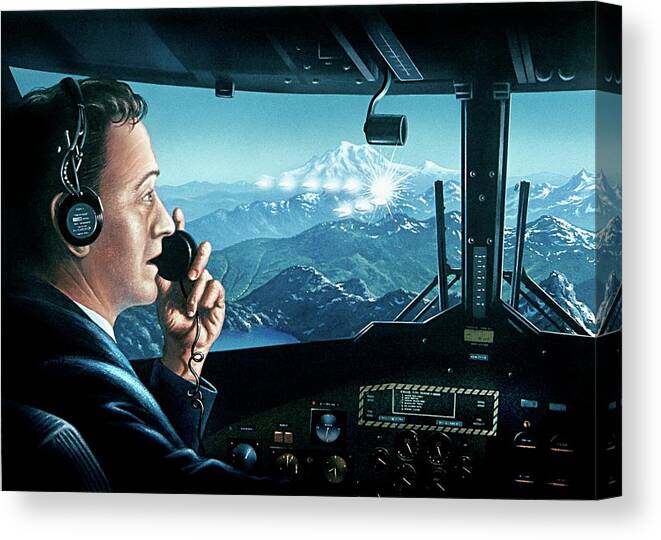This vibrant illustration depicts an older man, donning a dark suit with a white shirt, situated in the cockpit of a flying vehicle, likely a plane or helicopter. He has light skin, dark hair, and is wearing headphones while speaking into a handheld radio microphone. The detailed cockpit includes an array of black control panels and various buttons, as well as wiper blades on the windows. The scene through the two front windows reveals a bright, clear day with a vast expanse of bluish and white mountains, including a prominent snow-covered peak in the distance. Additionally, there are shiny objects in the sky that could be interpreted as UFOs and the glaring headlights of cars descending the mountainside, adding an intriguing sense of depth and activity to the picturesque landscape.